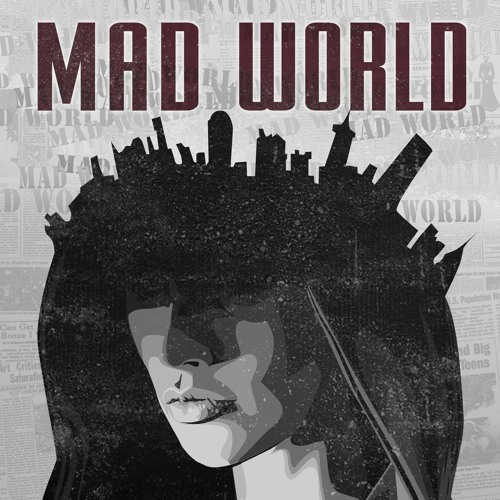This detailed image, possibly resembling an album cover or a poster, is titled "Mad World." It features a predominantly gray and dull background, which includes darkened phrases of "Mad World" across the top and throughout the backdrop, mimicking newspaper clippings and articles. Dominating the lower part of the composition is the silhouette of a woman's face, with her eyes obscured, her nose partly in shadow, and her closed lips leading down to her neck, all rendered in various shades of gray. Intricately integrated into her full, flowing black hair is a cityscape silhouette, where skyscrapers and buildings stretch from the left over the crown of her head to the right. Prominently displayed at the top in large maroon letters, the title "Mad World" contrasts against the subdued background, emphasizing the artwork's title and themes.